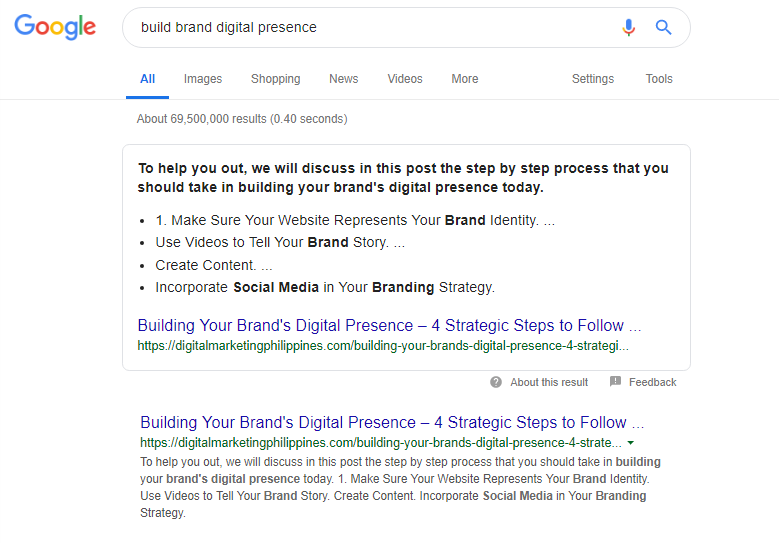Here is a detailed and cleaned-up caption for the provided image description:

---

The image shows a screenshot of the Google search results page. It is slightly wider than it is tall, set against an entirely white background. In the upper left corner, the Google logo is prominently displayed. Directly to the right is the Google search bar, which contains the text "build brand digital presence" in black. 

Below the search bar, a navigation menu is visible, showing the section options: "All" (highlighted in blue with an underline), "Images," "Shopping," "News," "Videos," "More," "Settings," and "Tools" (all in gray).

Underneath this menu, a brief line indicates that approximately 69,500,000 results were found in 0.4 seconds. Further down, there is a thin gray box containing a bolded statement: "To help you out, we will discuss in this post the step-by-step process that you should take in building your brand's digital presence today." This introductory text is followed by four bulleted points:

1. **Make sure your website represents your brand identity.**
2. **Use videos to tell your brand story.**
3. **Create content.**
4. **Incorporate social media in your branding strategy.**

At the bottom of this text box, a blue hyperlink reads, "build your brand's digital presence - four strategic steps to follow."

---

This cleaned-up caption provides a clear and detailed description of the image.